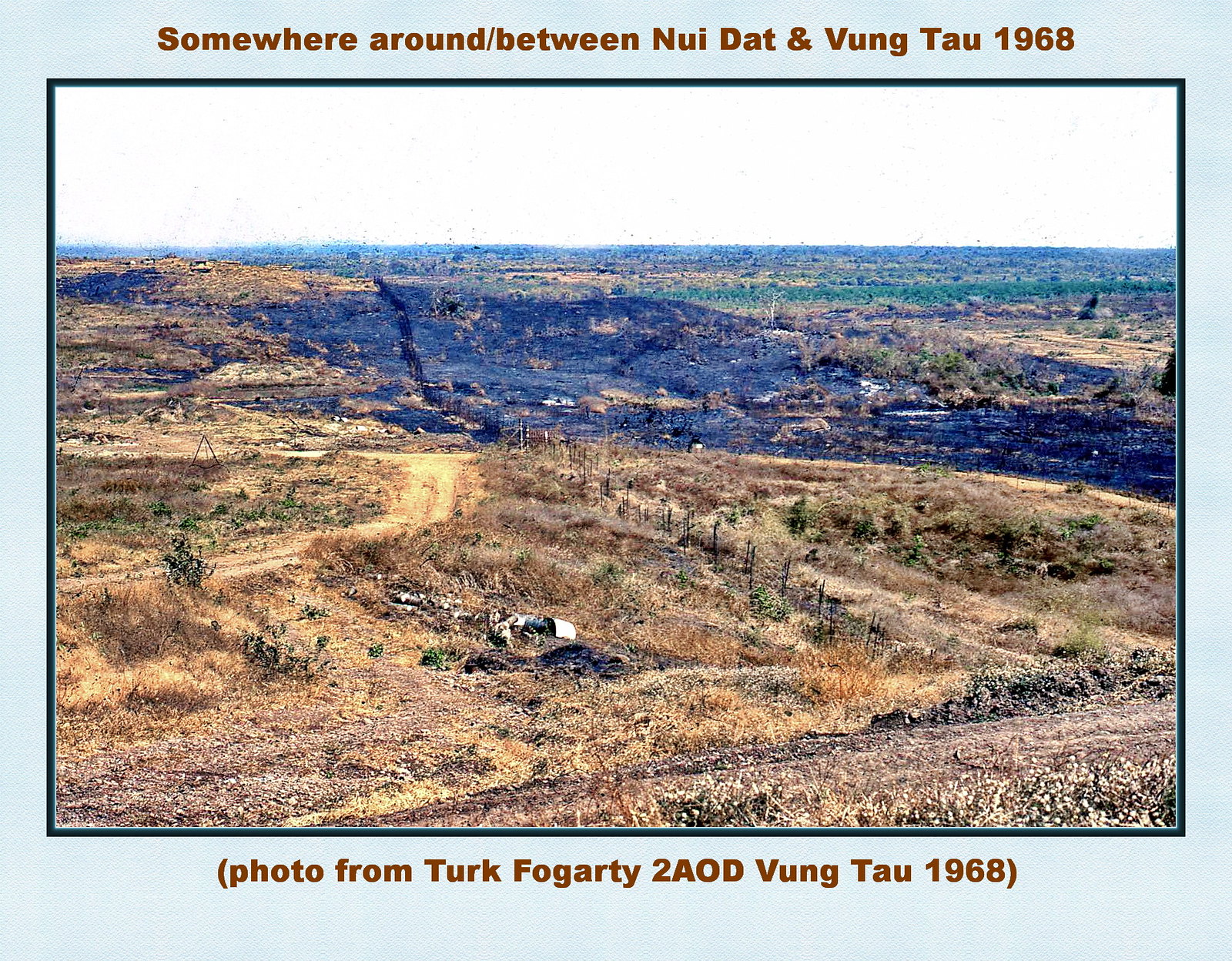This detailed photograph, reminiscent of an old postcard, is bordered by a dark blue frame set against a larger light blue rectangular background. Labeled at the top in brown font, it reads "somewhere around / between Nui Dat and Vung Tau 1968," while the bottom inscription states "photo from Turk Fogarty to AOD Vung Tau 1968." This image captures a sprawling rural landscape characterized by shallow hills and scrubby, short vegetation. A dirt road runs from the left side, winding through the scene. Dominating the foreground is a large, blackened, scorched area indicative of a recent fire, with patches of dark smoke still visible. The burnt path stretches from left to right, cutting through the vegetation. Beyond this scorched terrain, healthier, darker green vegetation can be seen in the distance, leading up to an overcast gray sky, additng a somber overtone to the overall setting. Small trees and shrubs are scattered throughout the horizon, enhancing the depth and bleakness of this historical landscape.